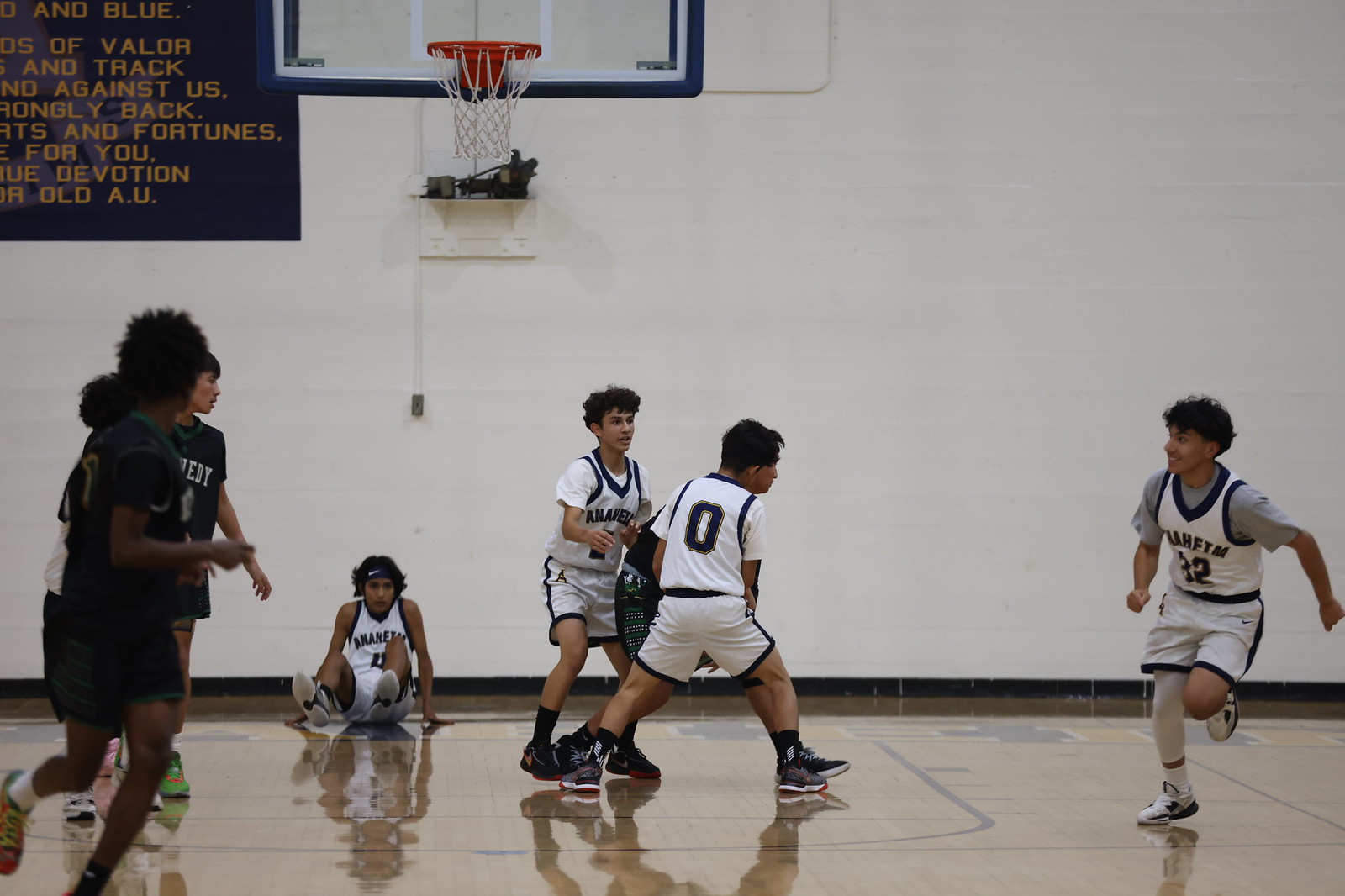This image captures a dynamic moment from a youth basketball game, likely involving players aged 13 to 14. The game is being played on an indoor court with white walls and a wooden floor. The photo is centered on a cluster of players vying intensely for the ball. The main action includes a player wearing a white jersey, possibly labeled "Anaheim" in blue letters with gold trim, and numbered 32. Another white-jerseyed player, numbered zero, has his back turned to the camera. Their opponents, in black jerseys with green trim, are also converging on the ball. There are a total of seven players visible: four in white and three in black. One boy, seemingly out of the play, is seated or has fallen out of bounds near the backboard. A basketball hoop is clearly visible against the white wall, and a banner with yellow letters on a black background hangs to its left, though most of the text is obscured. The intense scene suggests a fierce competition for ball possession.